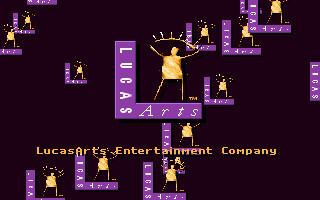In this intricately designed, computer-rendered image, the central focus is an emblematic "L" shape. The word "Lucas" runs vertically from the top to the bottom along the elongated vertical side of the "L," styled in bold print and oriented sideways. "Arts" is inscribed in italic print on the horizontal base of the "L." Rich in detail, the emblem features a gold outline of a person standing on the bottom part of the "L." Above this figure is a half-moon symbol with radiant gold lines emanating outward. Below this central emblem, the phrase "Lucas Arts Entertainment Company" is clearly centered, providing a definitive identification. The entire design is set against a stark black background, creating vibrant contrast. Additionally, various smaller renditions of the purple "L" shape, accompanied by the same gold figure, are scattered throughout the background in differing sizes and positions, adding depth and complexity to the visual composition.